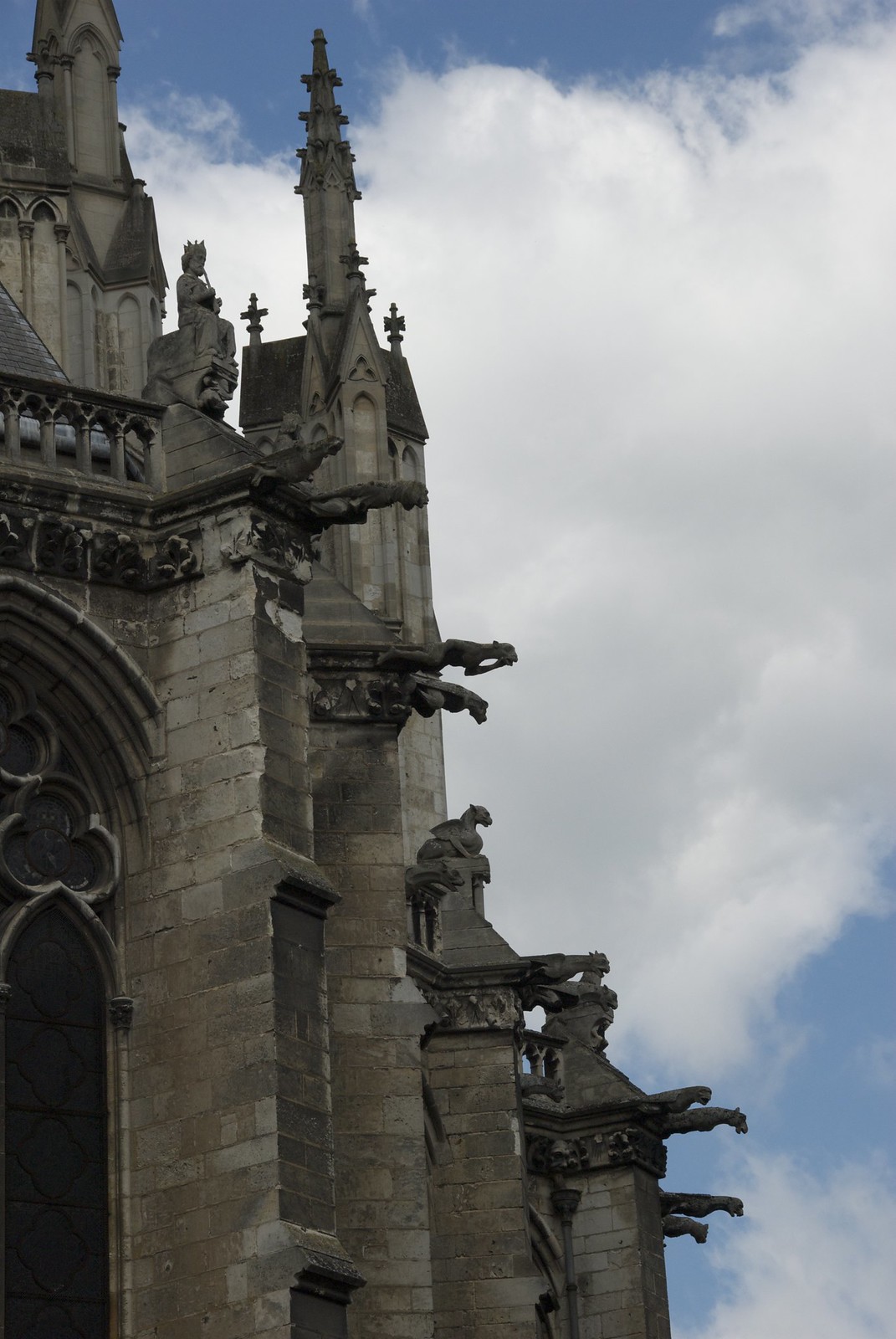This is a detailed photograph of an ancient, gray-stone cathedral, capturing its weathered grandeur from a unique, upward-facing angle. The cathedral, predominantly located on the left half of the image, features a stunning array of architectural details, including towering spires and numerous gargoyles jutting out horizontally from the structures, seemingly gazing down at viewers below. A prominent, tall, narrow window with a clover-shaped design at its apex is visible, adding to the building's medieval charm. The window appears almost completely black, contrasting sharply against the stonework. The edifice is adorned with intricate stone figures, including a king-like figure playing an instrument, animal-like creatures resembling leopards or sphinxes, and flying buttresses. Crosses atop the tower parapets further emphasize the religious significance of the structure. The backdrop features a serene blue sky dotted with large, fluffy clouds, enhancing the cathedral's majestic and timeless appearance.